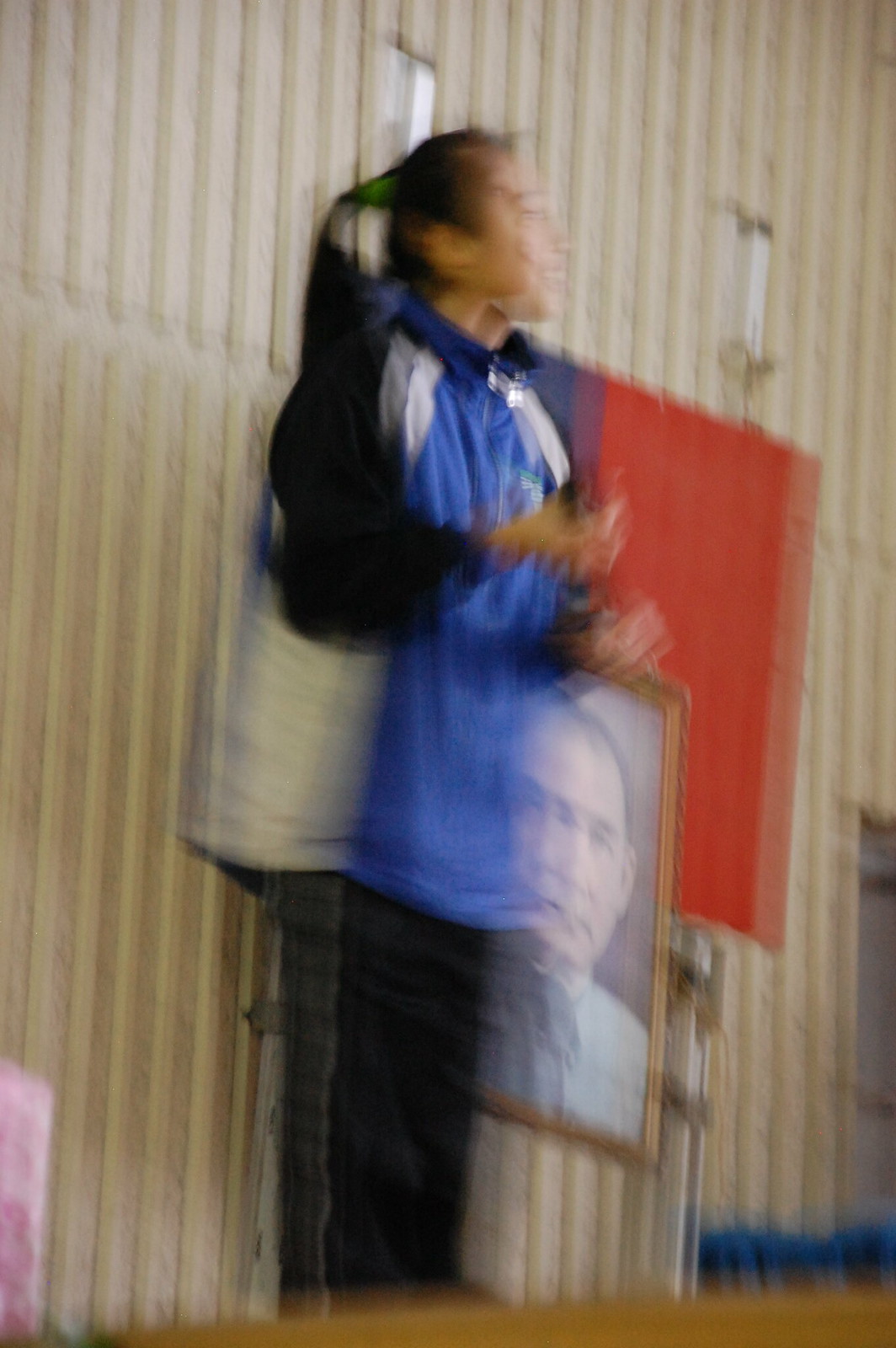In this very blurry photograph, a woman with black hair tied back into a ponytail with a green band stands in front of a tan ridged wall. She is wearing a distinctive blue and white zip-up coat with black sleeves, which is fully zipped up, paired with black and gray pants accented by a yellow line down the middle. Her skin has an olive complexion, and she appears to be Asian. She stands on a wooden podium with her hands raised and gazes off into the distance. To her right hangs a black and white portrait of a man with short dark hair, dressed in a light-colored shirt. The portrait is framed in gold and positioned against a backdrop featuring a black and red flag.